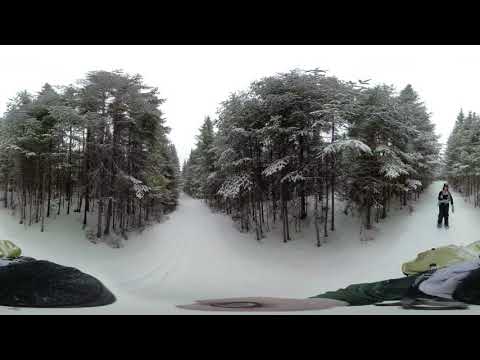This photograph captures a serene, snowy landscape featuring a scenic pathway cutting through tall, snow-capped trees, predominantly pine and birch. The pathway extends into the distance, flanked by rows of towering trees on either side. A person dressed in dark, long-sleeved clothes and black pants stands off to the right, nestled between the trees, adding a human element to the otherwise natural scene. The snow blankets the ground and the trees, giving them a glittering, dusted appearance. The sky is overcast and gray, lending a gloomy, yet tranquil ambiance to the scene. The image is framed by a half-inch thick black border at the top and bottom, and the overall photograph appears slightly skewed and blurred. An additional person can be vaguely seen holding the camera as if taking a selfie, though their details remain indistinct. The organized growth pattern of the trees adds a sense of orderly beauty to this wintry landscape.